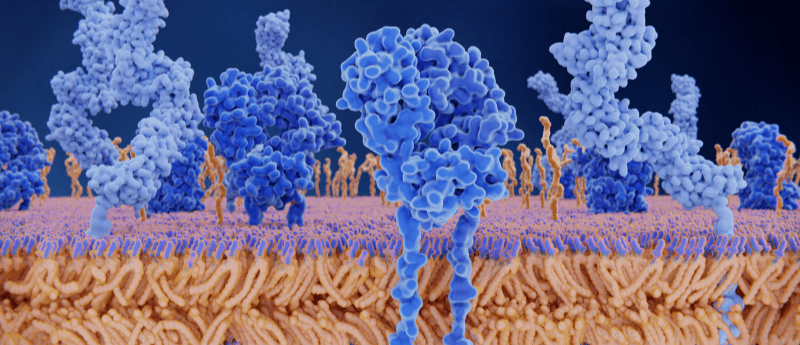The image is a detailed scientific illustration showcasing a cellular construct, possibly a cell membrane or phospholipids, set against a dark navy blue background. The primary focus is on two horizontal layers of cream-colored, thread-like structures that resemble the fibers of a shag carpet. These thread-like structures align to form an impression of legs, with their blue tips creating a solid blue surface towards the center. Interspersed among these layers are several clusters of irregular, pill-shaped globular structures in various shades of blue, with some extending into brownish, branch-like formations. The entire image gives the impression of a complex, microscopic world, blending an AI-generated aesthetic with photographic representationalism to elucidate receptors and their roles in cellular biology.